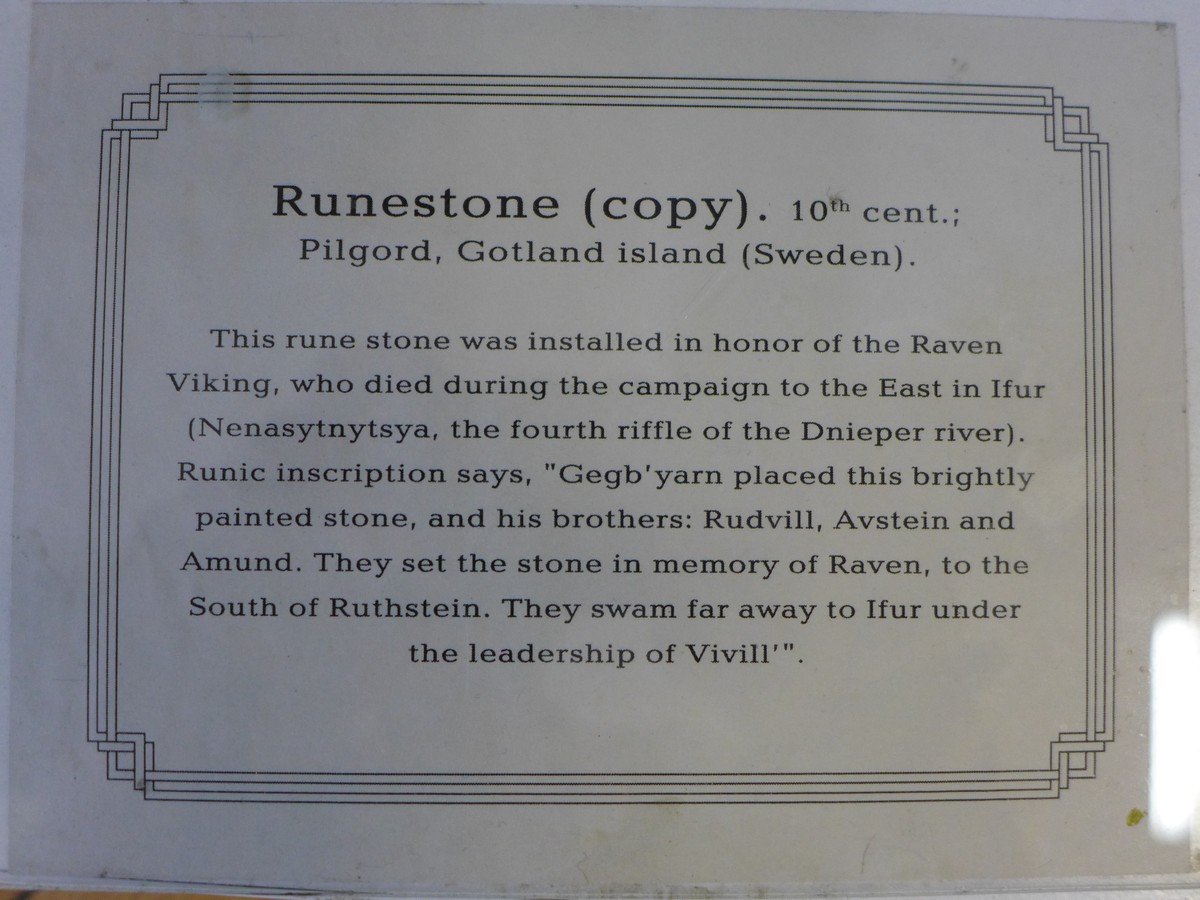The image shows a dark grey placard, possibly made of granite or cement, with a decorative edging framing the text. At the top, it prominently reads "Runestone (copy)." Below that, it identifies the artifact as from the 10th century and provides the location "Pilgored, Gotland Island, Sweden" in bold letters. The text explains that this runestone was installed in honor of the Raven Viking, who died during a campaign to the east in Eifur, Nenas-Tintisia, at the fourth riffle of the Dnieper River. The runic inscription notes that Gebjarn placed the brightly painted stone, along with his brothers Rudville, Avstein, and Amund, in memory of Raven to the south of Ruthstein. They ventured far to Eifur under the leadership of Vivel. The writing is black and bold, set against the grey background, with a line grid pattern accentuating the text.